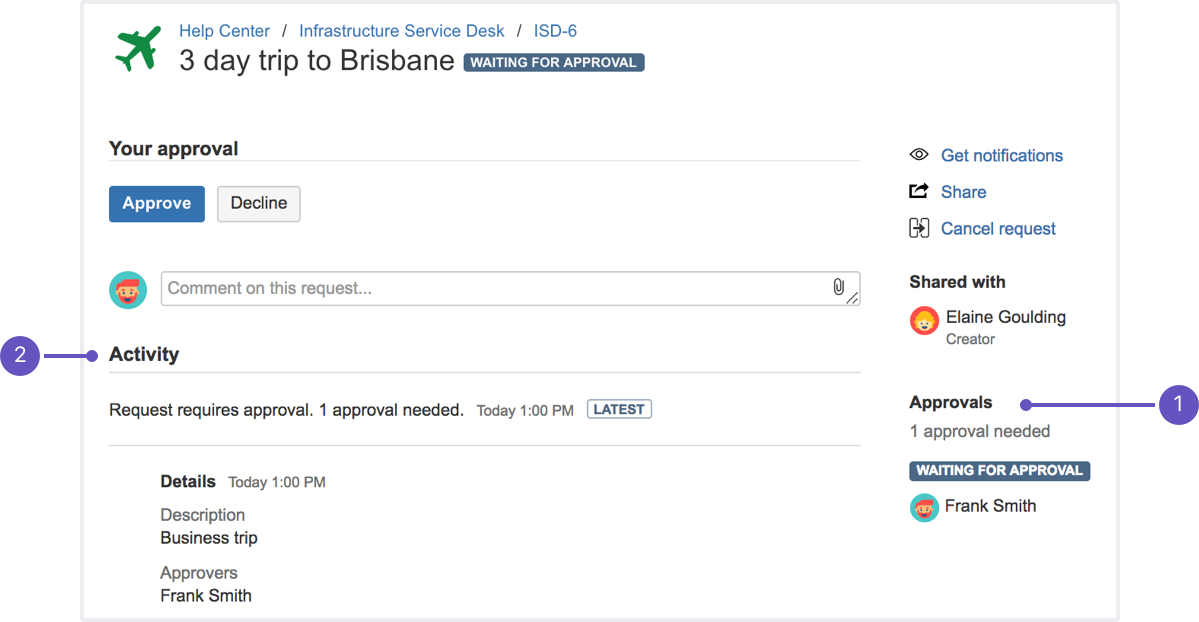A screenshot of a flight itinerary for a three-day business trip to Brisbane, displayed on an approval interface, likely part of a travel request program for a company. The page lacks any visible branding or indication of the website or app's name. The itinerary description is titled "Your Approval," followed by two prominent buttons at the bottom: a blue "Approve" button and a white "Decline" button. There is an empty text field allowing the user to enter comments on the request. Below this field, a menu labeled "Activity" shows a notification that the request requires approval, with one approval needed by 1 p.m. today. Additional details provided include the nature of the trip ("business trip"), the approver ("Frank Smith"), and the collaborator ("Alain Golding").